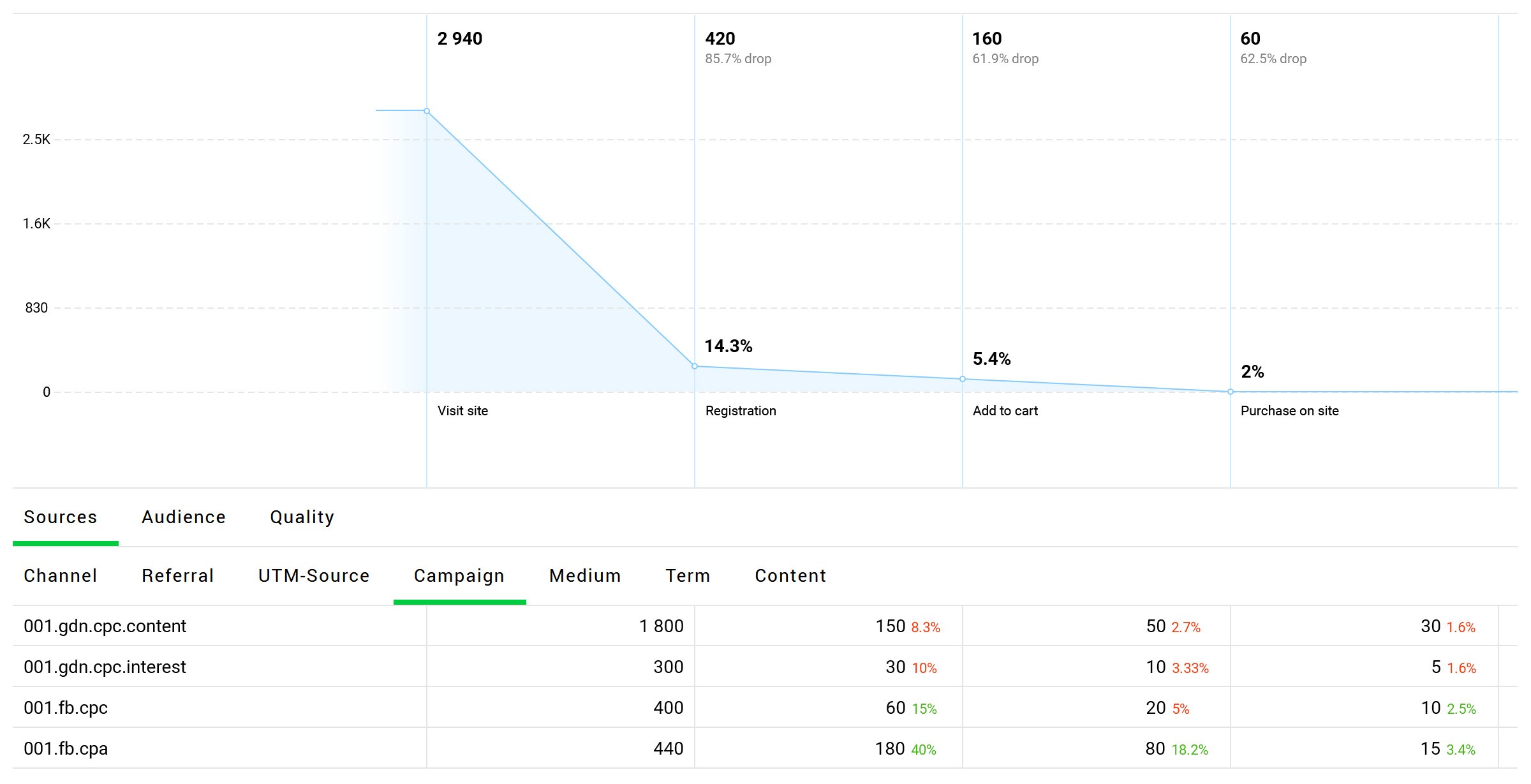The image features a detailed analytical graph set against a solid white background. The vertical axis on the left is labeled with numerical values: 2,500, 1,600, 830, and 0. The horizontal axis to the right is categorized by stages of site interaction: "Visit Site," "Registration," "Add to Cart," and "Purchase on Site." 

Below these stages, there is a breakdown of various sources: "Sources," "Channel 001," "GDN," "CPC.Content," with respective values: "Term 1,800" and "Content 150." Additionally, it specifies other key metrics like "Sources," "Audience," and "Quality."

Further down, different tracking parameters are listed, highlighted with a green underline: "Channel," "Referral," "UTM Source," "Campaign," "Medium," "Term," and "Content." Specific data points follow: "001.GDN.CPC.Interest" shows 300 visits, with subsequent registrations at 30, items added to the cart at 10, and final purchases at 5.

This meticulous breakdown provides a comprehensive view of visitor interactions and key performance indicators across various marketing channels and stages of the purchase funnel.